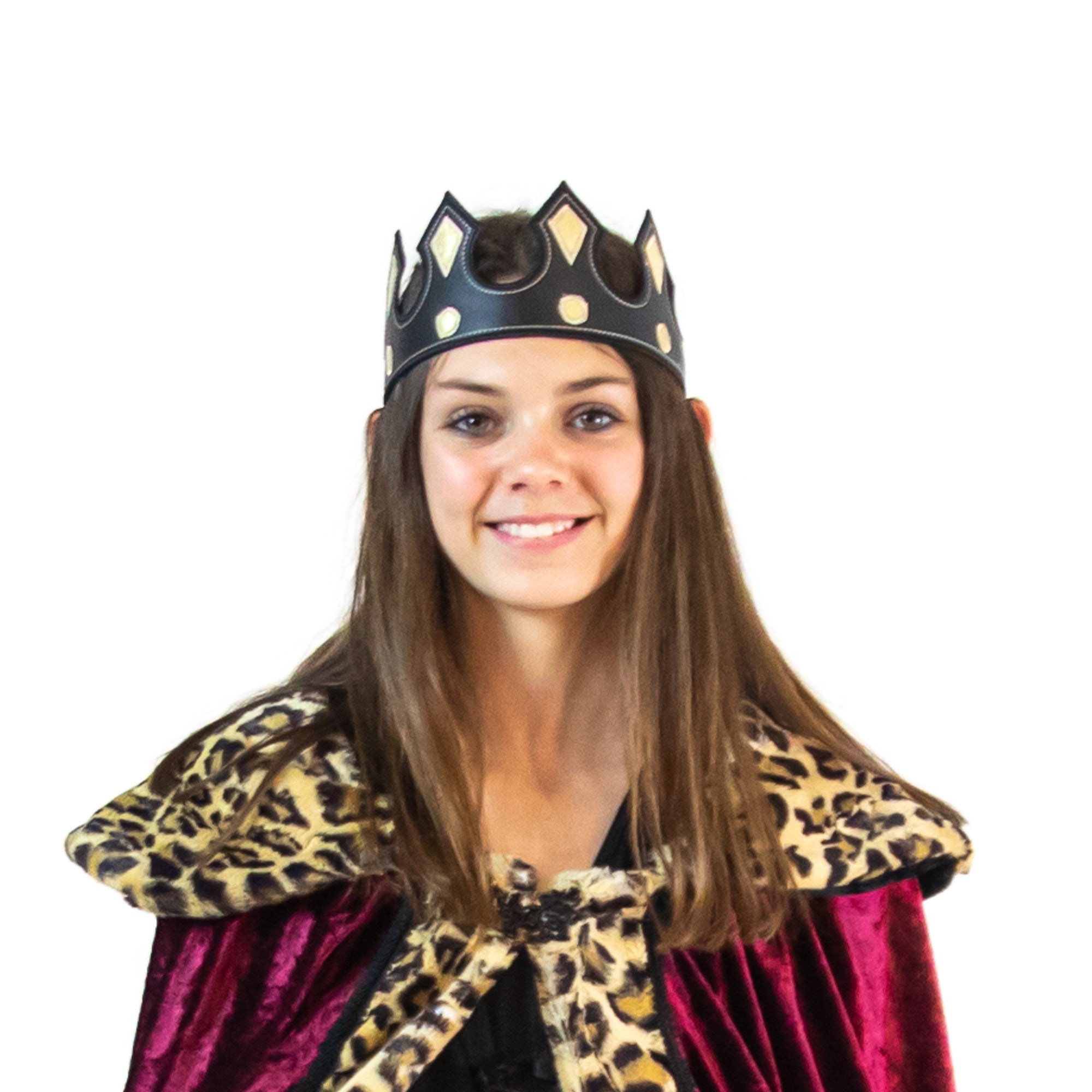The image is a full-color, staged photograph of a young Caucasian woman, likely in her late teens to mid-twenties, standing against a plain white background with no text or watermarks. The focus is on her costume, which suggests she is dressed as a queen for a costume event. She has long, straight brown hair cascading down to her chest, and striking blue eyes. Her smile is warm and inviting.

She is adorned with a black crown embellished with goldish-yellow diamonds, and her outfit consists of a deep maroon or purple velvet robe. The robe is trimmed with faux leopard skin fur along the shoulders and down the front. Underneath the robe, she wears a black shirt, although only the top portion of her outfit is visible. The detailed textures and colors of her costume, along with her cheerful expression, create a vivid and engaging image.